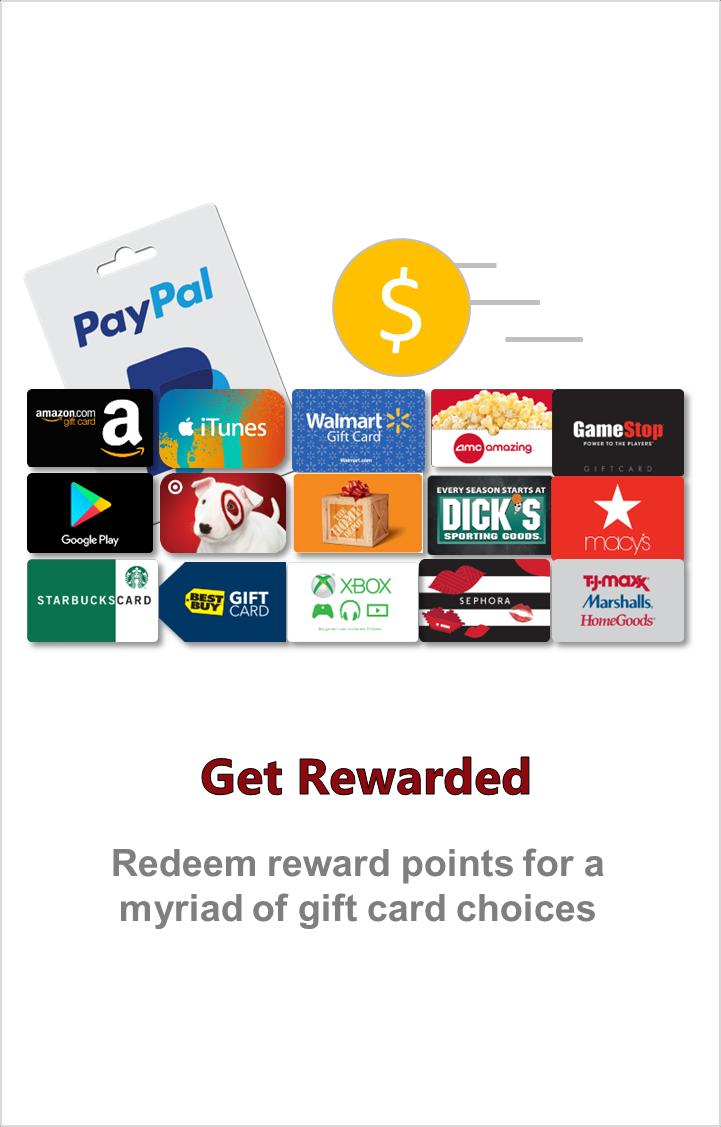This vibrant, color screenshot from a website features a clean, white background with an arranged array of various gift cards and currency methods at the top. A distinctive PayPal card in grey, partially obscured and positioned at an angle, peeks out from behind the other cards. Beside it, a symbol representing Bitcoin—a yellow circle adorned with an 'S'—is visible, though the accompanying small black text is illegible.

Among the prominently displayed gift cards are those for popular retailers and services, including Amazon, iTunes, Walmart, KFC, Camel shop, game shop, Google Play, and several others. Notably, there are also gift cards for a pet-themed shop, one depicted with a box, DICKS, Macy's, Starbucks, Best Buy, an unidentified card, Xbox, Sephora with its distinctive stripes and petals design, TK Maxx, Marshalls, and Home Goods.

Directly below this assortment, the text "Get Rewarded" is displayed in a dark brown hue. Beneath it, a black font elaborates with the phrase, "Redeem reward points for a myriad of gift card choices." This caption underscores the diverse options available, highlighting over 12 choices including PayPal, Bitcoin, and a combination card usable across TK Maxx, Marshalls, and Home Goods.